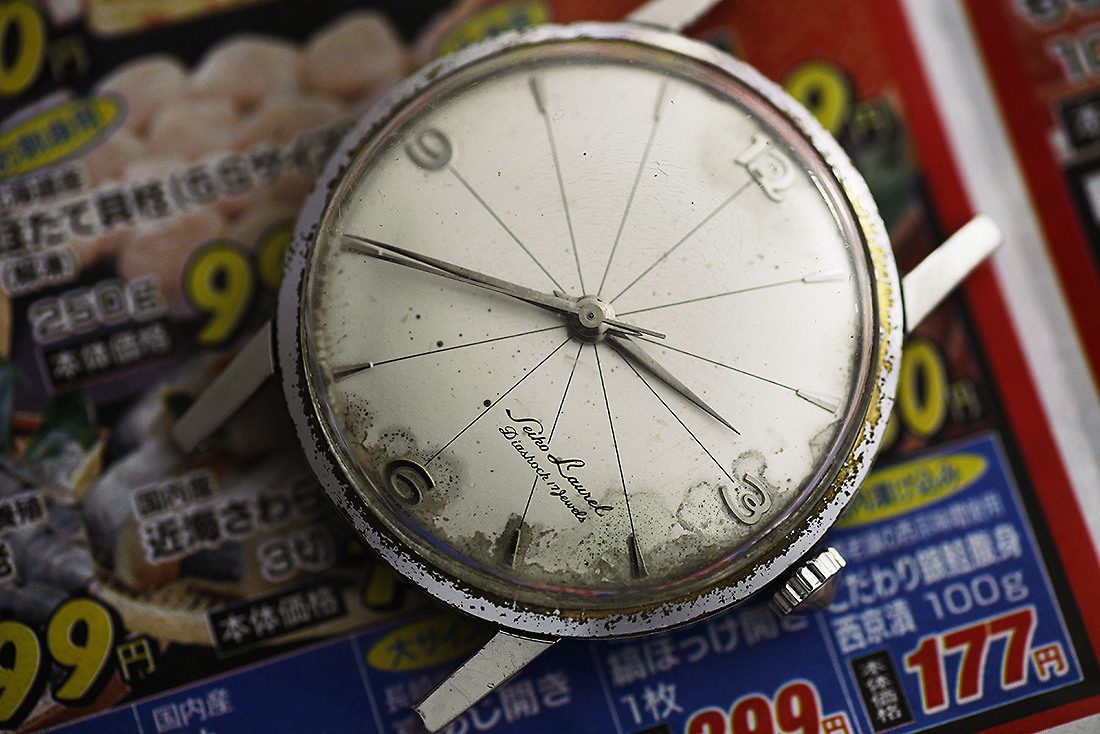The image features a timeworn wristwatch, noticeably lacking its original strap but retaining its band holders. The watch's chrome exterior exhibits signs of wear and tear, suggesting it has endured extensive use over the years. The dial is minimalist, marked only by the numerals 12, 3, 6, and 9, while the remaining hour indicators are represented by understated lines. The overall impression is that of a vintage timepiece with a rich history evident in its visible imperfections and aged appearance.